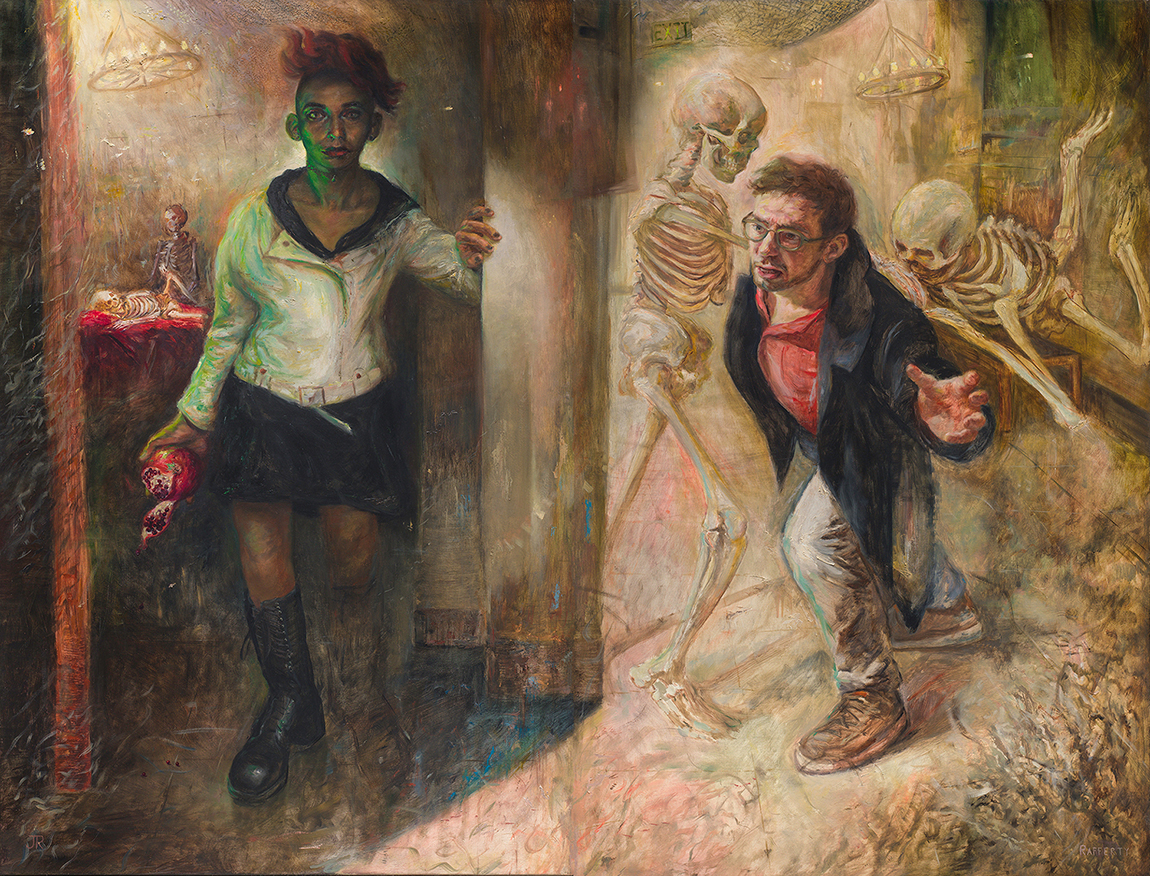This color painting, titled "Persephone and Hermes in the Underworld," by Jason Albert Rafferty from 2019, is a modern surrealist work in landscape orientation. The image is detailed and thought-provoking. It depicts a woman standing on the left side of the image and a man on the right, both separated by a partition of a wall section.

The woman on the left has dark skin and long hair piled on top of her head. She is dressed in a white jacket, a black mini skirt, and black thigh-high boots. In her right hand, she holds a half-eaten pomegranate. There is also a suggestion that she might be missing a leg, holding something that appears bloody, which adds an eerie dimension to the scene. Behind her is a doorway leading to a table with a red tablecloth where a skeleton is seated.

On the right side, the man appears to be lunging forward on his left knee as if peering around the corner. He is dressed in beige pants, leather boots, a dark jacket, and a red polo shirt. His appearance includes gray or brown hair. Surrounding him are skeletons, with one standing next to him and another hanging from the wall. There is also a chandelier with lights hanging above, illuminating the scene.

The melding of the surreal elements with the classical myth of Persephone and Hermes creates a haunting and enigmatic atmosphere, making this artwork a captivating piece to decipher.